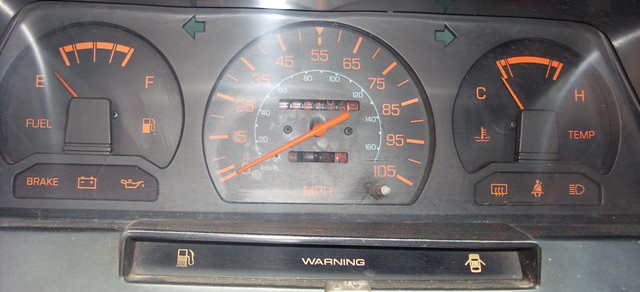The image captures a close-up of a car dashboard, though the make and model of the vehicle are indeterminate. At the bottom of the frame is a small bar that protrudes slightly, displaying a series of indicators. On the left side of this bar is a gas gauge icon, marking the location of the fuel tank. Adjacent to this, on the right, is an icon of a car with its doors open. Centrally located in this section is the word "WARNING," and the entire area appears to be coated with a layer of dust.

To the upper left, there is a fuel gauge, which currently indicates that the tank is empty, though it's likely that the car is not turned on or in motion. Embedded within the fuel gauge, to the right, is a small icon of a gas pump, signifying which side of the vehicle the fuel door is on. Below this area, the words "BRAKE," "BATTERY," and "OIL" are legible, suggesting that these are status indicators for various checks.

To the right and slightly above this section is the left-turn signal arrow. Next to it is the speedometer, marked with bright orange numerals, ranging from 0 to 105, and a prominently colored needle. The odometer is also visible but obscured by glare, making the reading indiscernible. Adjacent to the speedometer is a temperature gauge, completing the array of monitoring instruments.